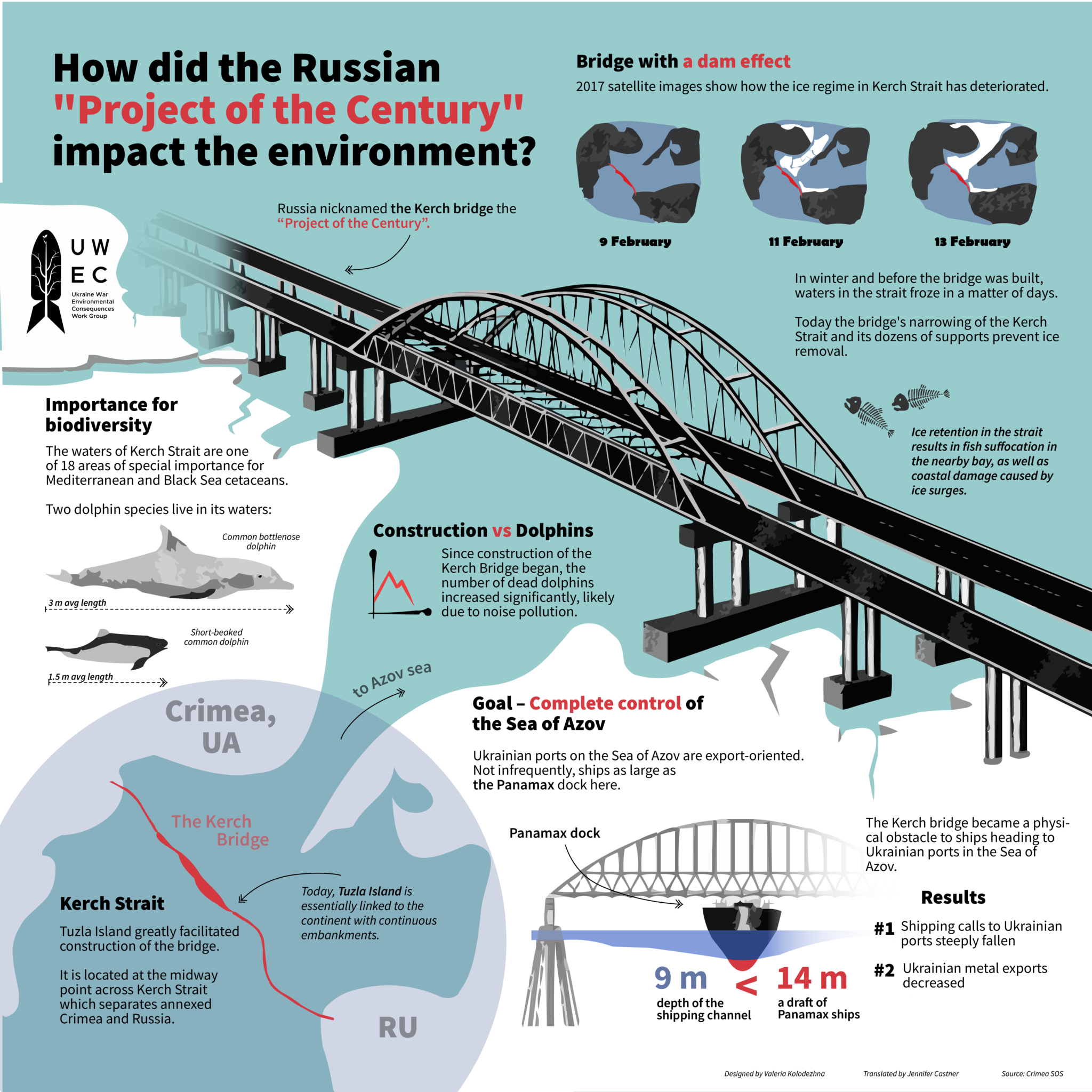The infographic, set against a bright blue background, centers on the question, "How did the Russian Project of the Century impact the environment?" highlighted in black and red font in the upper left corner. The image prominently features a detailed diagram of the Kerch Bridge spanning diagonally from left to right. On the upper right, it discusses the "Brent with the Dam Effect, 2017," illustrating how the ice regime in the Kerch Strait has deteriorated with three satellite images from February. It states that before the bridge's construction, the strait's waters froze rapidly during winter, but now, the bridge's numerous supports impede ice formation.

In the bottom-left section, the infographic emphasizes the "Importance for Biodiversity," noting that the Kerch Strait is one of 18 critical areas for Mediterranean and Black Sea cetaceans. It highlights the presence of two dolphin species: the common bottlenose dolphin and the short-beaked common dolphin. The section "Construction vs. Dolphins" reveals a significant increase in dolphin deaths since the bridge's construction, likely due to noise pollution.

The bottom text mentions the geopolitical aspects, stating that the bridge connects annexed Crimea and Russia via Tuzla Island, which facilitated the construction process. Today, Tuzla Island is linked to the continent through continuous embankments. Additionally, it notes the goal of achieving complete control over the Sea of Azov, affecting Ukrainian ports and their export capabilities.

Overall, the infographic conveys the environmental and geopolitical impacts of the Kerch Bridge project, combining ecological concerns with strategic motives.